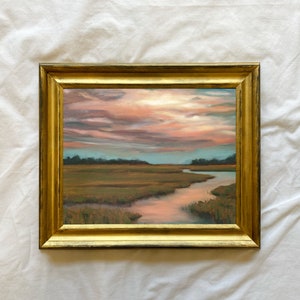This image showcases a detailed painting taken from above, set against a white fabric backdrop that features noticeable folds, suggesting the painting is not mounted on a wall. Enclosed in a three-tiered gold wooden frame, the artwork illustrates a tranquil scene of a flat, grassy wetland or inlet with a meandering river reflecting the sunset, giving the water a pinkish hue. The land around the river is a mix of brownish tones, and the background boasts a lush gathering of distant trees and shrubs reminiscent of a forest. Above, the sky transitions from blue to a canopy of beautiful white and pinkish cirrus clouds, creating a serene and picturesque landscape devoid of human presence.